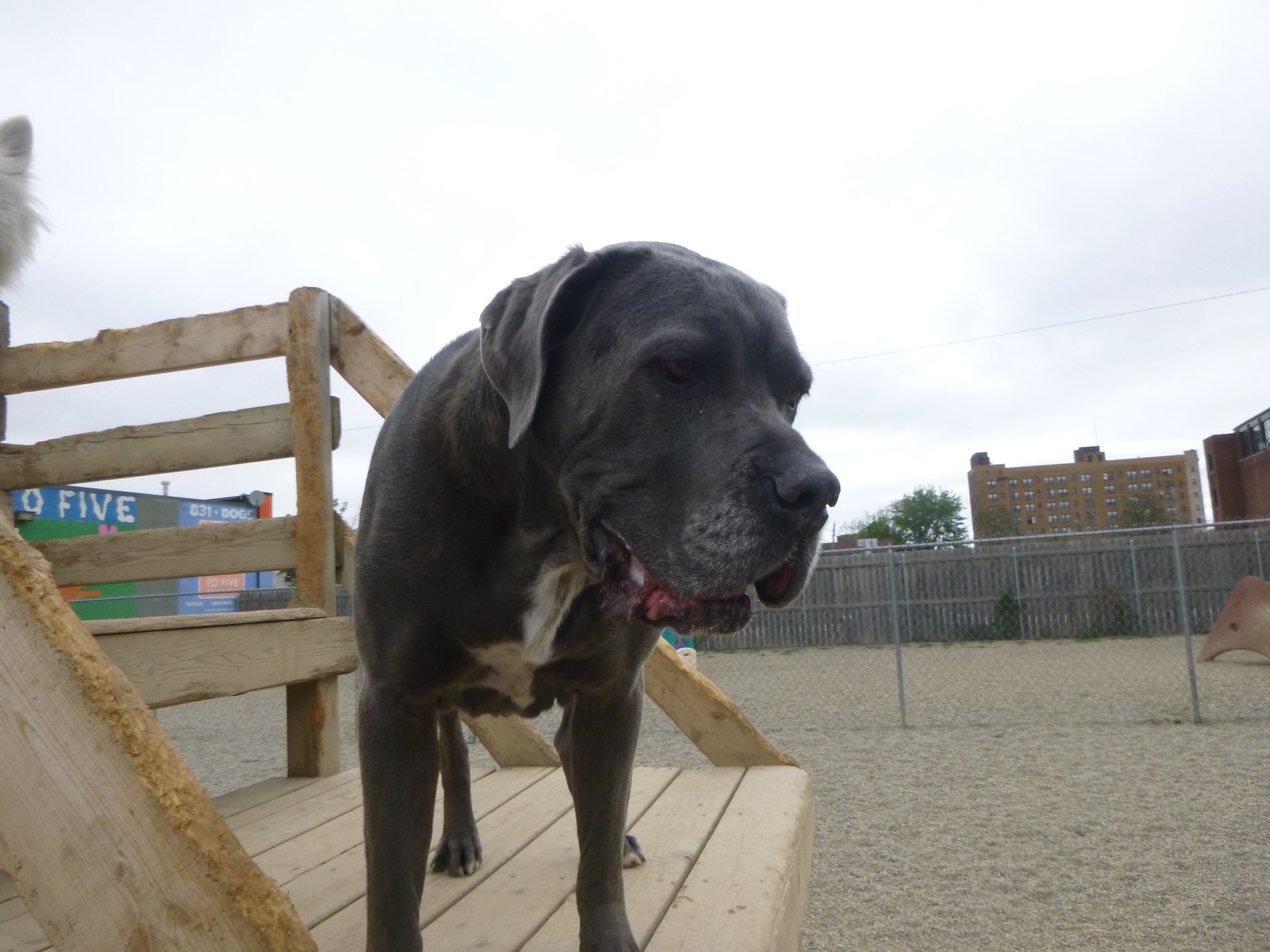In this image, we see a large, mostly black dog, possibly a crossbreed with a face resembling a bloodhound. The dog's nose, eyes, and slightly open mouth are visible as he looks almost directly at us. He has a white patch on his belly and his ears are down. The dog is standing on what appears to be a wooden step or part of a boardwalk in a fenced play area with white sand beneath. In the background, there are multiple layers of fences: a metal chain-link fence followed by a heavier, opaque fence, suggesting another play area. Further in the distance, there's a tree and an overcast sky. To the left, we see a tall red building, possibly an eight to ten-story residential structure with many small windows. Additionally, there is another building visible on the left side with a phone number partially painted on it, suggesting "something 5-F-I-V-E." The scene seems to be a mix of natural and urban elements, blending a playful environment for the dog with the surrounding high-rise structures.